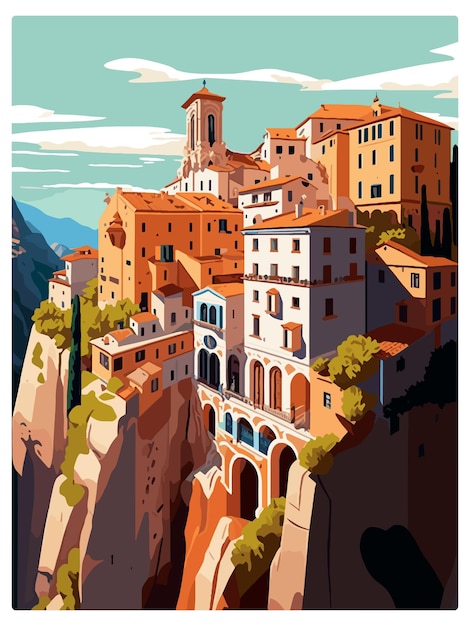This detailed illustration depicts a quaint village, resembling those found in Italy or Greece, perched precariously on the cliffs of a mountainous terrain. The art style is reminiscent of a paint-by-numbers painting, with a slightly flat and cartoonish aesthetic, rich in vibrant and contrasting colors. The overall palette is dominated by shades of rusted yellow, light olive green, and terracotta, with blue and teal hues for the sky.

The village consists of tightly-packed buildings, many of which are interconnected. Predominantly, the buildings are painted white, sandstone pink, and a range of warm tones including light yellow and terracotta. They have ornate facades with rounded doors and windows, some with blue shutters, while others have painted decorations and small balconies. Several structures, especially the rooftops, are gold-colored, reminiscent of terracotta tiles. Among the buildings, a prominent church with a stone steeple and gargoyle carvings stands out, towering above the rest.

The lower levels of the buildings feature wooden arched entries, characteristic of Mediterranean architecture. Below these houses, there are sheer rock cliffs with patches of grassy vegetation clinging to their edges. The cliffs are interspersed with cylindrical trees and pale olive green plants. An additional structure that resembles an aqueduct with arched formations is visible, adding to the classic European charm.

In the background, there are shadowed mountain peaks in shades of gray and blue, contributing to the picturesque and serene landscape. The sky is a soft teal blue, adorned with delicate, wispy white clouds, completing this idyllic scene of a hillside village nestled in nature's embrace.